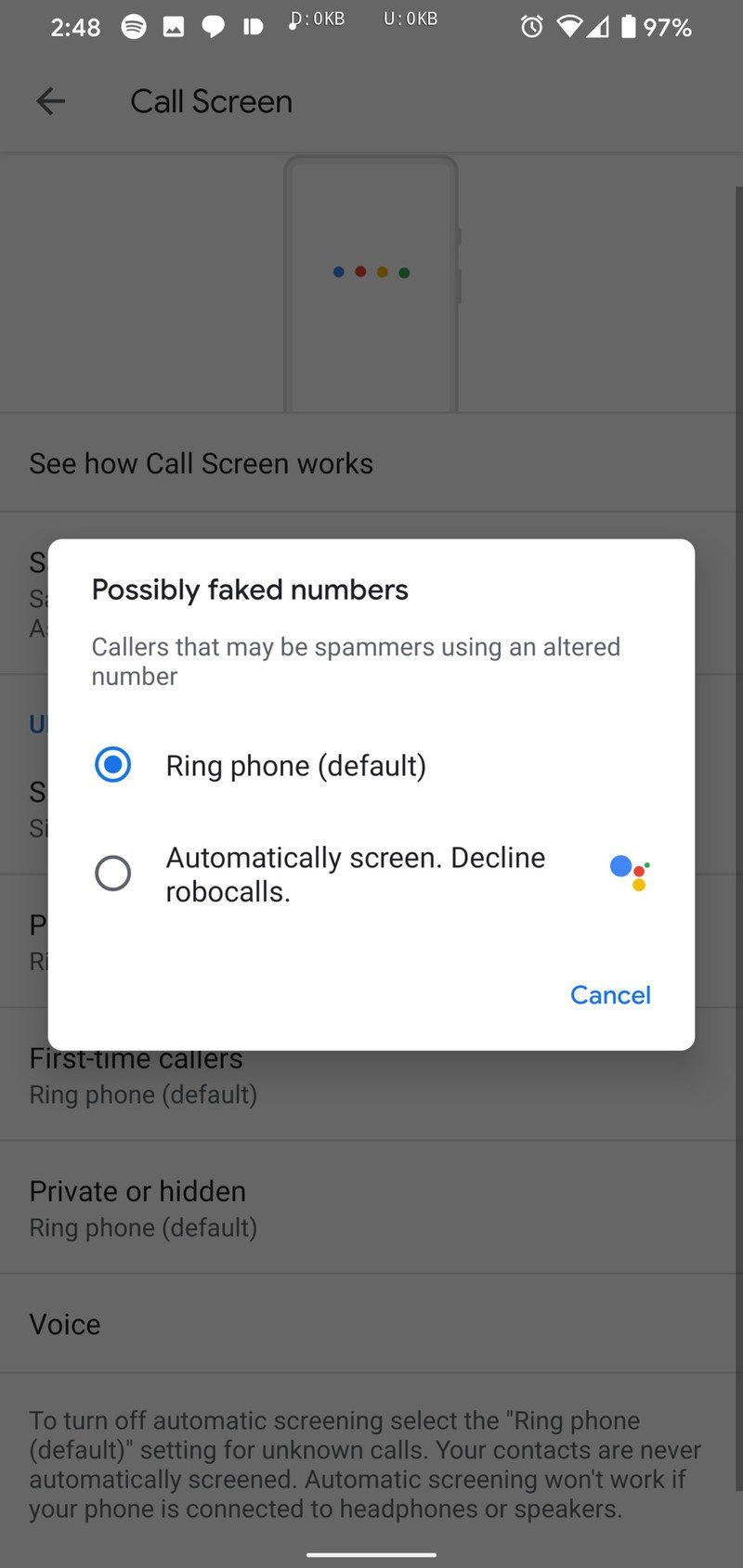The image is a screenshot of a smartphone's call screen interface. It displays an alert indicating that the incoming number might be a "possibly faked number." The app further explains that such numbers are often used by spammers who alter their caller ID. 

The interface offers two response options:
1. "Ring Phone," which is the default setting, as indicated by the blue circle.
2. "Automatically Screen and Decline Robo Calls."

Additionally, there is a "Cancel" button at the bottom of the pop-up window. The background screen behind the alert is grey and features various sections titled "Call Screen," "How Call Screen Works," "Private or Hidden," "Voice, First Time Callers," among other notifications.

In the status bar at the top of the screen, it's visible that the phone's battery is at 97%, the alarm is set, and the screenshot was captured at 2:48 PM. Also, the Spotify app is active.